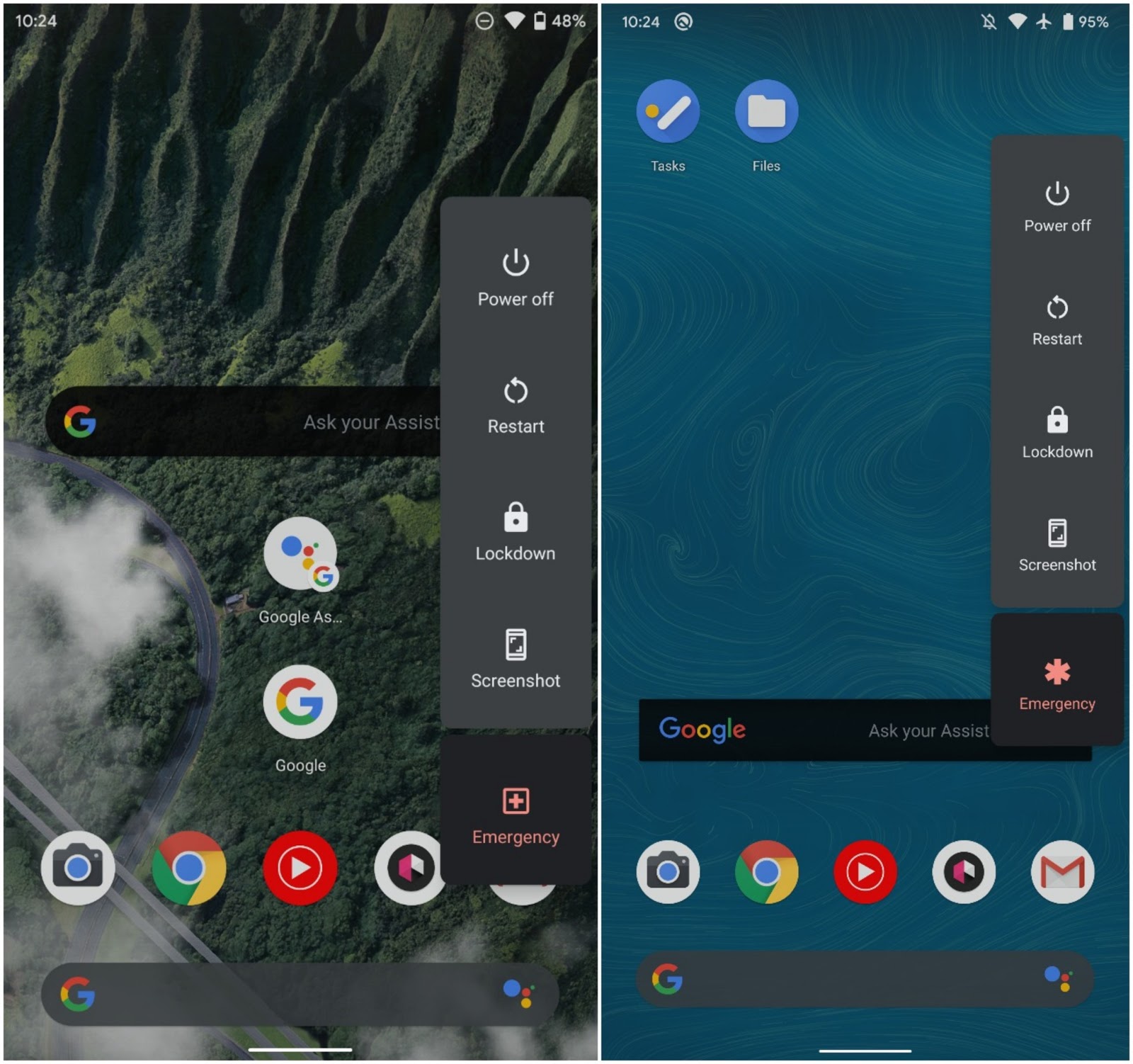The image consists of two side-by-side screenshots from cell phones. The screenshot on the left depicts an aerial view, showcasing a landscape with a dense cluster of trees occupying the lower half. In the bottom left corner of this image, there appears to be either clouds or smoke. The upper portion reveals a tall, mountainous cliff. Above this image, a Google bar is displayed, featuring the iconic Google 'G' and various function bubbles, including the Google Play symbol, the camera, Chrome, a play button, and a search bar at the bottom.

The screenshot on the right presents a visual of swirling blue water mixed with dynamic white swirls. In the upper left corner, there are two blue circles, one labeled 'Tasks' with an icon resembling a stick and ball, and another labeled 'Files' with a white folder icon. Lower down, there is a black bar with the Google logo. Similar to the left screenshot, the bottom is populated by multiple icons including the camera, Chrome, a red play button, and the Gmail 'M'.